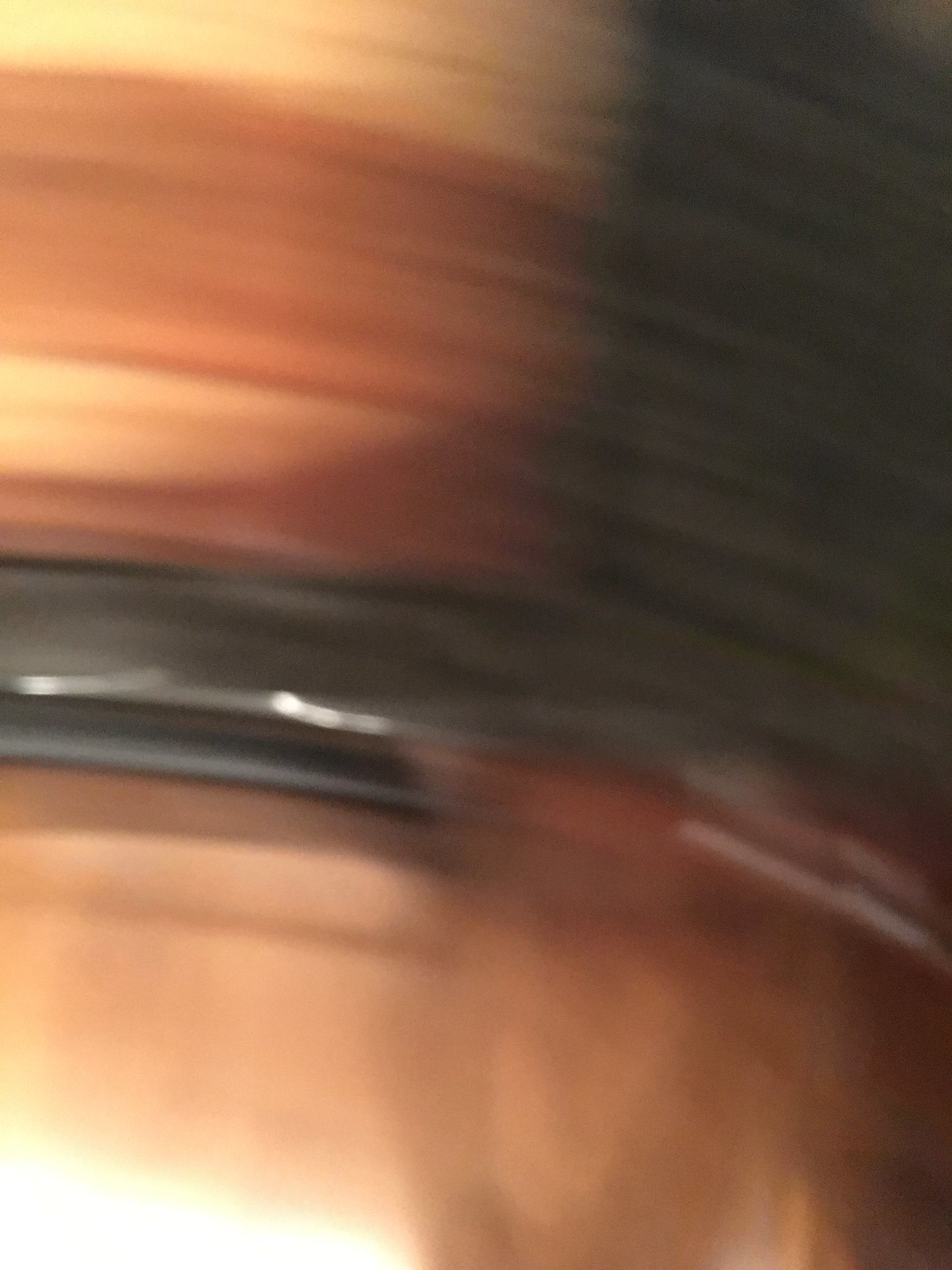A heavily blurred image capturing an abstract and ambiguous scene, featuring a gradient of brown hues at both the top and bottom. White stripes intersect the composition, while a prominent gray ring with a hint of reflective light slices through the center. The upper portion of the scene is deeply shadowed, creating a stark contrast with the patterned middle section, which includes alternating bands of white, brown, and black. A glaringly bright white light emerges from the bottom left corner, adding a sharp focal point. The image evokes the appearance of a close-up view of a celestial body, reminiscent of Saturn or Jupiter, or alternatively, the intricate interior of a clay ceramic vase.